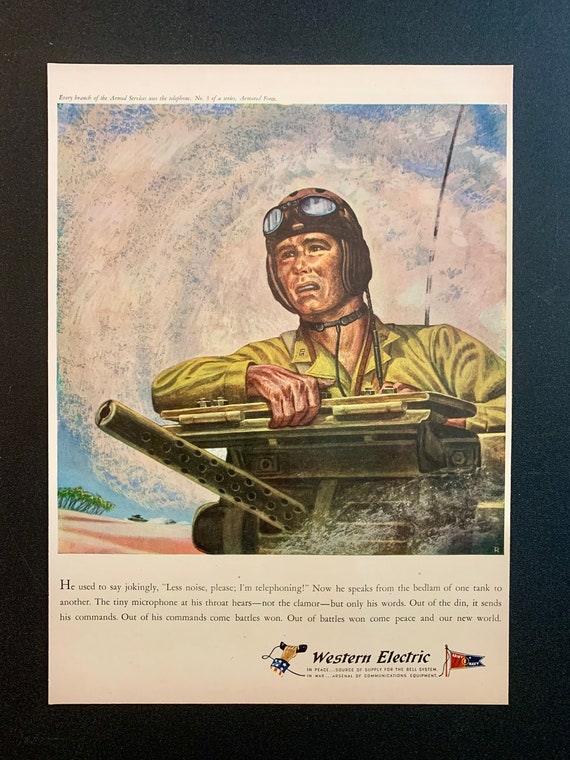The image is a detailed photograph of a World War II-era advertising poster for Western Electric, set against a bluish-black background reminiscent of an art gallery display. The poster, with a lithographic style, features a GI prominently in aviation gear—including a pilot's helmet and goggles on his forehead—suggesting his involvement in both communication and combat. Clad in a green or lime green shirt, the GI appears to be manning a tank-mounted machine gun, gazing determinedly into the distance. The scene behind him includes a blue sky filled with swirling white clouds or jet trails, creating a dynamic backdrop. In the far distance, additional tanks can be faintly discerned, adding to the wartime atmosphere. Below the illustration, a narrative extolls the virtues of Western Electric's communication technology, attributing battlefield success and eventual peace to the clear commands transmitted by a tiny microphone at the GI's throat. The Western Electric logo and cursive text are prominently featured at the bottom right, adding an official branding touch to the historical advertisement.